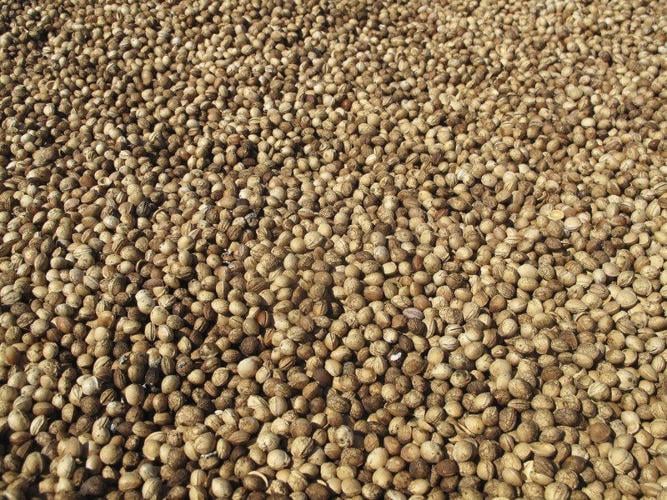This landscape-style photograph captures an endless expanse of what appears to be pistachio nuts, piled high and extending beyond the frame, suggesting an industrial-level production. The nuts, approximately the size of a pea, vary slightly in color from light tan to dark brown, but overall present a uniformly brownish tint. Some of the pistachios are open while others remain closed, adding to the texture and detail of the image. The focus is sharper in the foreground, particularly in the upper bottom left corner, gradually blurring into the distance, emphasizing the sheer volume and continuity of the pistachio pile. Despite the slight variations and high-resolution clarity, the image maintains a cohesive and visually overwhelming sea of these nuts, revealing no other elements or distractions.